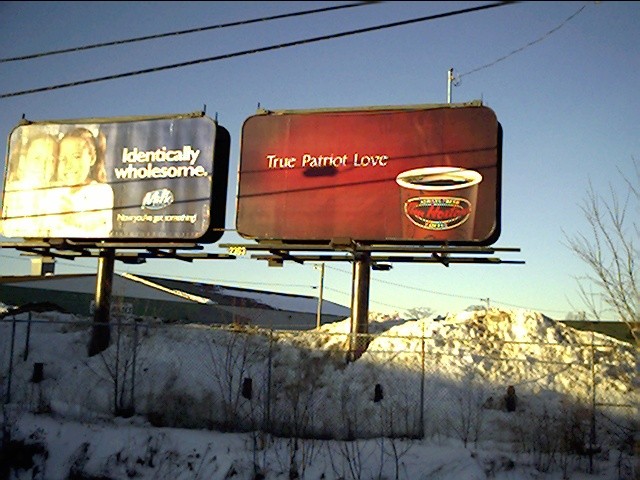This slightly rectangular, horizontal image captures a striking winter scene featuring two side-by-side billboards set against a backdrop of snow-covered ground. The billboards, identical in shape and size, stand prominently in a pile of snow. Behind them is a long, wide building with a dark roof. The stark winter landscape is further accentuated by leafless trees positioned to the right of the image. A clear blue sky stretches above, contrasted by two visible power lines in the upper left corner.

The foreground is dominated by a snow-covered ground, bordered by a fence that runs across the lower portion of the image. The left billboard displays a duo of twins against a black background with white text that reads, "Identically Wholesome." Below this, it suggests, "Now you've got something." The right billboard stands out with its vibrant red background and a cup of coffee positioned on the lower right side. White text on this billboard proclaims, "True Patriot Love."